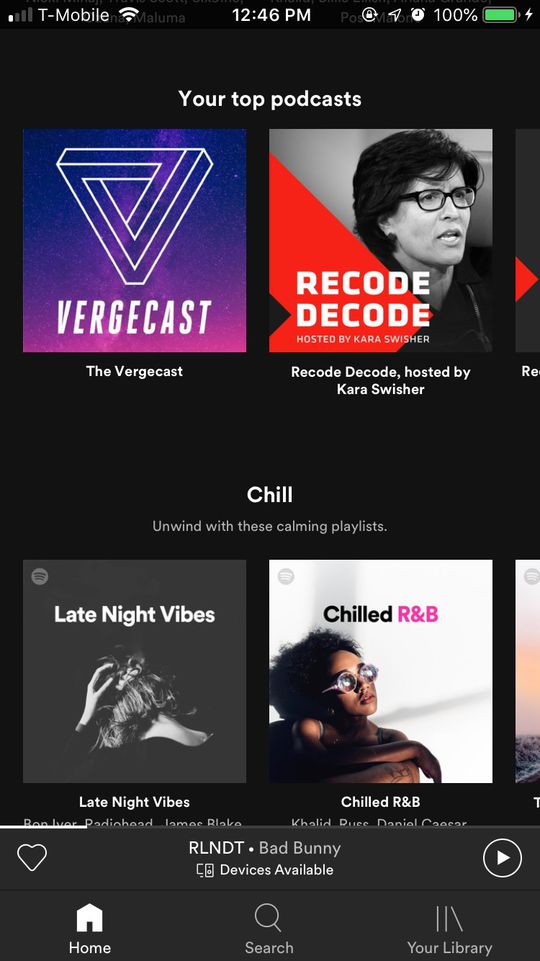Here is a detailed and cleaned-up descriptive caption of the image:

---

The screenshot depicts a podcast application interface with a black background. In the status bar at the top of the screen, there is one signal bar illuminated out of four on the upper left corner, indicating service strength. Next to it, the carrier name "T-Mobile" is displayed. To the right of the carrier name, there are three full Wi-Fi bars. At the center lies the current time, 12:46 p.m. Moving further to the right, there is an icon of a lock encircled by an arrow, indicating the screen rotation lock is active. Adjacent to this is the location services icon, then an alarm clock icon, followed by a "100%" label indicating battery life. Finally, there is a green battery icon with a white lightning bolt, indicating the device is plugged in and charging.

Below the status bar, the text "Your Top Podcasts" is prominently displayed in white. Under this heading, two podcasts are visible. The first podcast is titled "The Vergecast," and it features a cover with a blue and purple background, along with a white triangle and text. The title "Vergecast" is clearly displayed on the cover. The second podcast is "Recode Decode, hosted by Kara Swisher," featuring a black and white image of Kara Swisher. Kara has brunette, short hair styled to cover her ears and extending slightly down her neck. She's wearing black glasses and appears to be speaking. Next to her, a red triangular line partially overlays the image, with bold white capital letters stating "Recode Decode, hosted by Kara Swisher."

Below these podcast listings is the label "Chill," accompanied by the subtext in gray, "Unwind with these calming playlists." Two playlists are visible in this section. The first playlist is titled "Late Night Vibes," with a black and white cover showing a woman undoing her hair clip. The second playlist, "Chilled R&B," has a white background and features a black woman relaxing with natural light shining on her. She is wearing black round glasses. The title "Chilled" is in black text, and "R&B" is in red text.

At the bottom of the screen is a menu bar. In the center of the menu is a heart icon labeled "RLNDT Bad Bunny Devices Available." To its right is a play button icon. Below this row, there are three more icons: a home icon, a search icon, and a "Your Library" icon, for additional navigation within the application.

---